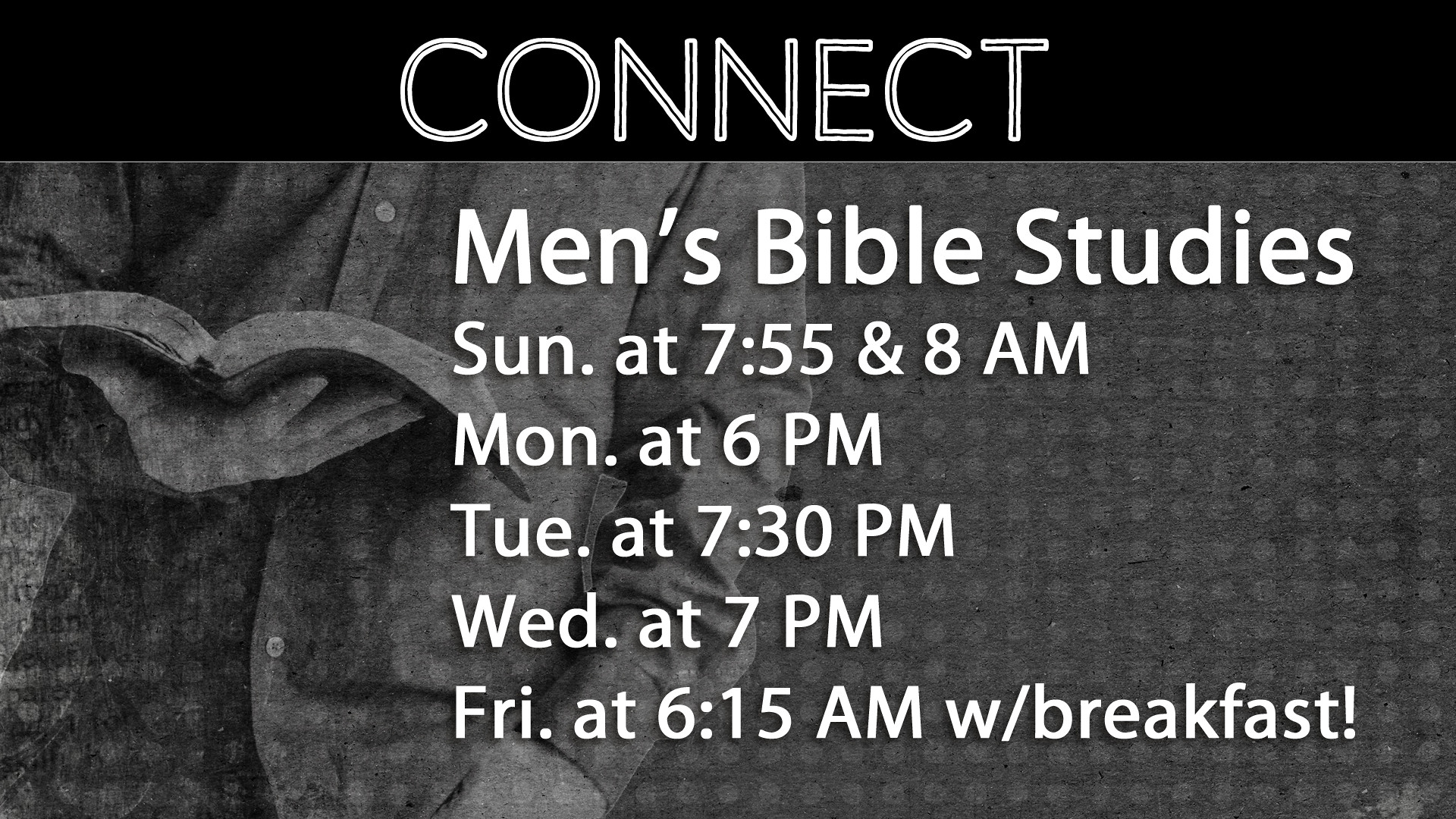This image features a slide with a graphic design style. The slide has a dark aesthetic, starting with a black banner at the top where the word "CONNECT" is prominently displayed in bold, white, all-caps text. Below this banner, the background is a faded, grey depiction of a person's torso grasping an open Bible, highlighted with soft, white polka dots. Superimposed over this background, in clear white text, it reads:

"Men's Bible Studies
Sunday at 7:55 AM and 8:00 AM
Monday at 6:00 PM
Tuesday at 7:30 PM
Wednesday at 7:00 PM
Friday at 6:15 AM with breakfast"

Overall, the design blends a spiritual theme with practical information, emphasizing connectivity and religious study.